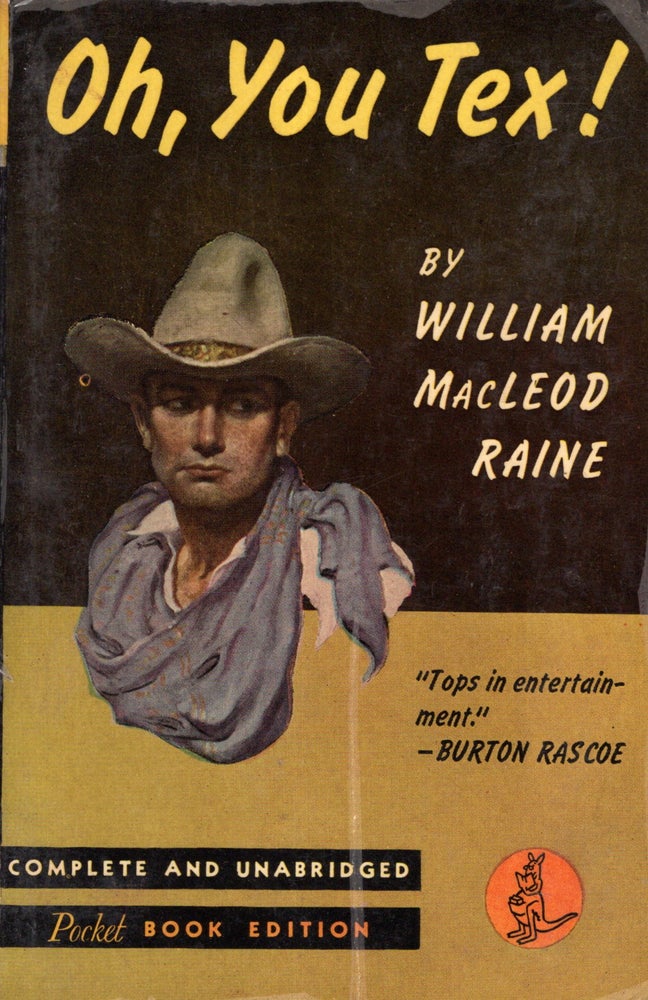This is an image of a vintage pocket book edition cover featuring a man in cowboy attire at its center. The background transitions from a dark brown at the top to a lighter tan-brown at the bottom. At the very top, bold yellow letters spell out "OU!" followed by "By William McLeod Raine" prominently displayed to the right of the cowboy figure. The cowboy, wearing a gray hat with a gold band, a white shirt, and a sash around his neck, is clean-shaven and positioned centrally on the cover.

Below the cowboy image, the background color shifts to a brown, where multiple black text boxes are arranged. The first black box contains the text "Complete and Unabridged" in white. The second black box features the words "Pocket Book Edition" in a subtle orange hue. Along the right side of the brown section, it reads "Tops in Entertainment" followed by a line and the name "Burton Rascoe."

At the very bottom of the cover, there is an orange circle containing a drawing of a kangaroo with a baby in its pouch, adding a unique touch to this vintage cover design.